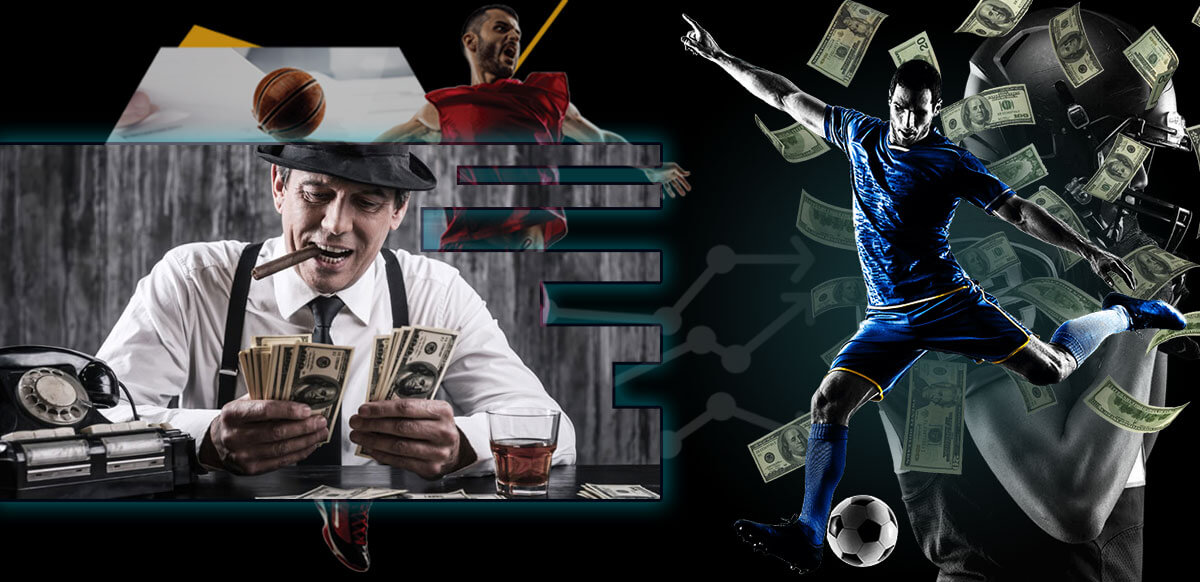In this long, rectangular, two-part image collage, the left side features a man who appears to be a bookie. He is dressed in a white long-sleeved shirt with suspenders, a black tie, and a black hat with a brim. He has a cigar in his mouth and is counting $100 bills on a green table beside an old, tiny, black rotary phone and a drink in a glass. Above him, integrated into the photo, is an anime character in the top right corner. On the far right side, there's a soccer player, wearing a blue jersey, blue shorts, blue socks, and blue and black shoes, caught in mid-action as he kicks a soccer ball. Scattered $100 bills can also be seen floating around in the background. Additionally, the background features the partial arm of another man, adding a layered, blended effect to the entire scene.